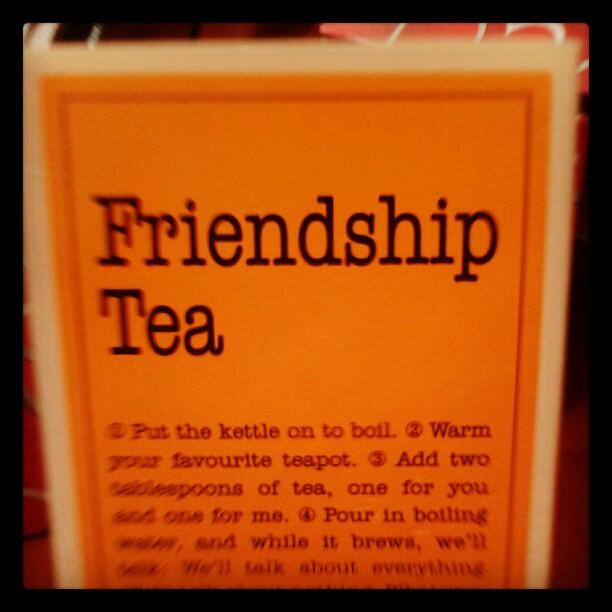This close-up image features a bright orange card with a white border and a thin black outline. The main focus of the card is the bold, black text that reads "Friendship Tea" at the top. Below this title, the card provides a set of instructions, partially visible due to the blurry and cut-off sections. The readable part of the text says: "Put the kettle on to boil. Warm your favorite teapot. Add two tablespoons of tea, one for you and one for me. Pour in boiling water, and while it brews, we'll talk. We'll talk about everything." The rest of the instructions are obscured, but it is clear that these steps are meant to facilitate a shared tea experience. In the background of the image, there are indistinct red, white, and black lines, possibly indicating another part of the book or background pattern, which contrasts with the simplicity and warm tone of the Friendship Tea card.